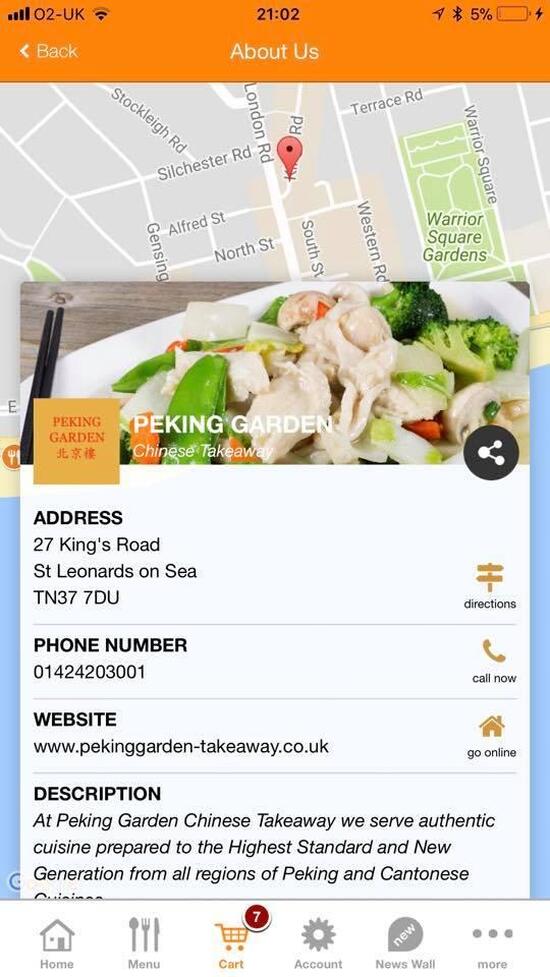The image shows a cell phone screen featuring an app, likely for ordering food from a restaurant. At the top of the screen, the status bar indicates it’s connected to “02-UK” with active Wi-Fi, showing the time as 21:02 and a critically low battery level at 5%.

On the main part of the screen, there’s a map that displays the location of "Peking Garden, Chinese Takeaway" situated at 27 Kings Road, St. Leonards-on-Sea, TN37 7DU. Above the map, the restaurant’s name is prominently displayed twice. To the right of the address, there are options for directions and a phone number (014-242-03001), along with a "Call Now" button for direct contact.

Below this, additional information and navigation options are available: 
- The website link for the restaurant (pekinggarden-takeaway.co.uk) 
- An option to "Go to online"
- A brief, cutoff description indicating that Peking Garden serves authentic cuisine from Peking and Cantonese regions, prepared to the highest standards.

At the bottom of the screen, several icons are visible:
- A home icon symbolized by a house.
- A menus icon represented by a fork, knife, and spoon.
- A shopping cart icon showing there are 7 items in it, indicated by a red circle with a white number seven.
- An account icon denoted by a gear cog.

Overall, the screen provides detailed information and options for ordering food from Peking Garden, a Chinese takeaway restaurant.